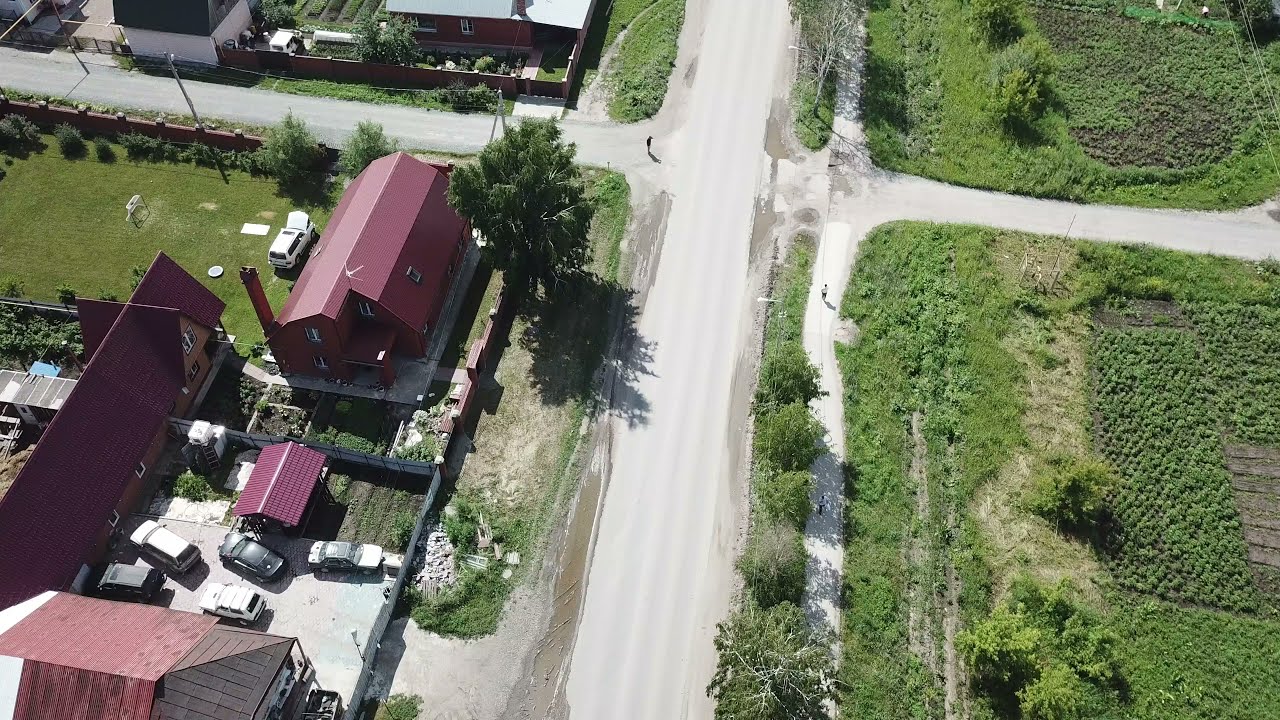This aerial photograph, likely taken from a drone or aircraft a few hundred feet above ground, captures a sunlit intersection of two gravel roads set at slight diagonals, with the wider road running vertically and the narrower one horizontally across the top of the image. Shadows cast by trees and bushes indicate clear skies. The vertical road is flanked by distinct features: on the right, green fields and a garden area dotted with bushes, and on the left, several houses, most notable for their red roofs. One house, prominent for its barn-like shape with a pronounced roofline, stands out among the structures, which include another building with a sharply angled roof, resembling a church or a garage.

Towards the center-left of the intersection, a figure is visible standing in the middle of the vertical road, while another person is near a pathway that runs parallel to this road, close to the intersection. The residential area features lawns and driveways with a total of five cars parked, including one in a fenced or garaged area. The intersection itself lacks stop signs, underscoring the rural or semi-rural nature of the setting. This image offers a detailed snapshot of a tranquil neighborhood, juxtaposed against verdant fields and structured homesteads.